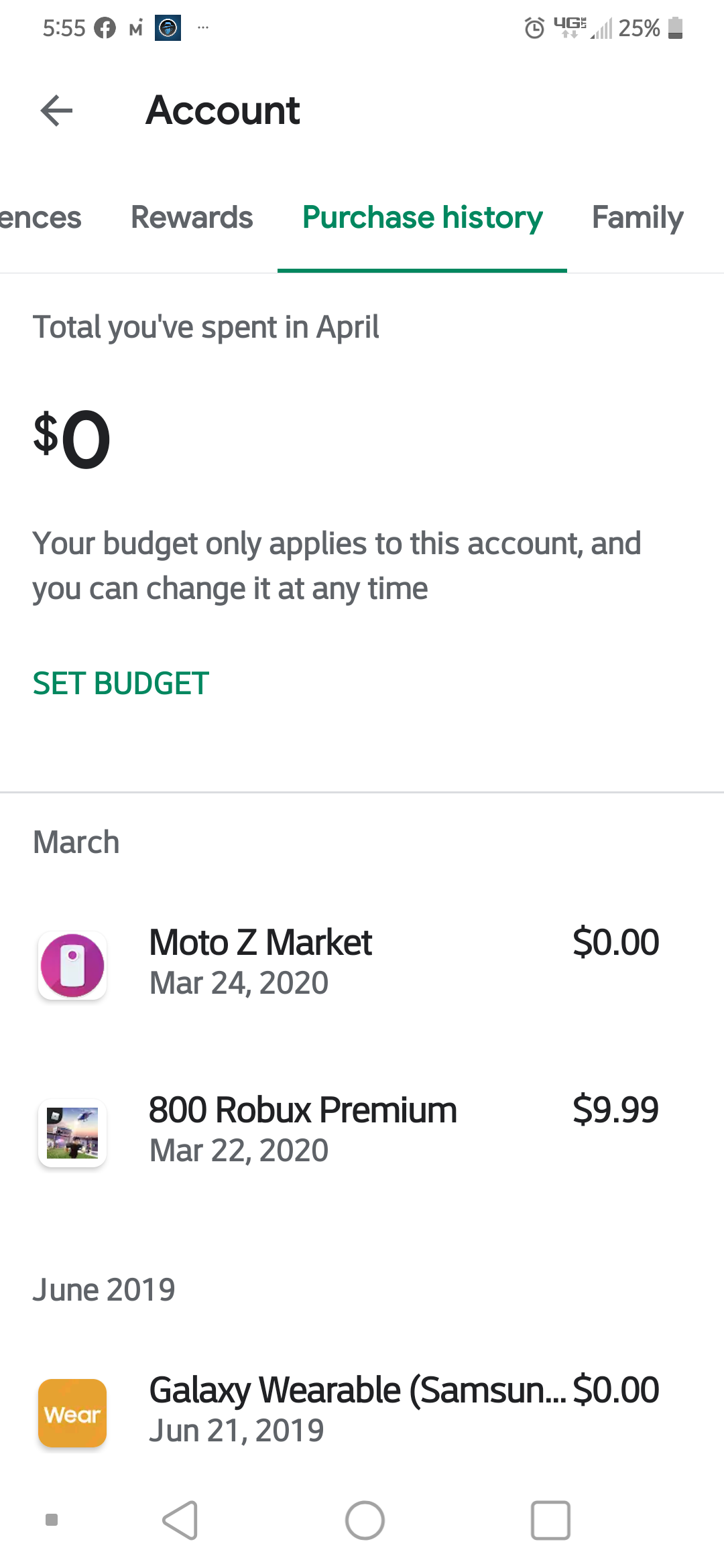This screenshot displays a mobile app's account summary screen. At the top of the screen, the heading "Account" is prominently displayed. Below this, there are several tabs: "Rewards," "Purchase History," and "Family."

Beneath these tabs, there is a section labeled "Total You Spent in April." It indicates that no money was spent in April ("$0"). A note explains that the budget applies only to this specific account and can be modified at any time, with an option to set a budget.

Following this, the app outlines spending details for different months. Under the "March" section, it shows an entry for "Moto Z Market," with a cost of $0. Another entry lists "800 Robux Premium" with a cost of $99.

In the "June 2019" section, there is an entry for "Galaxy Wearable" with the vendor noted as "Samsung" and the date specified as June 21, 2019.